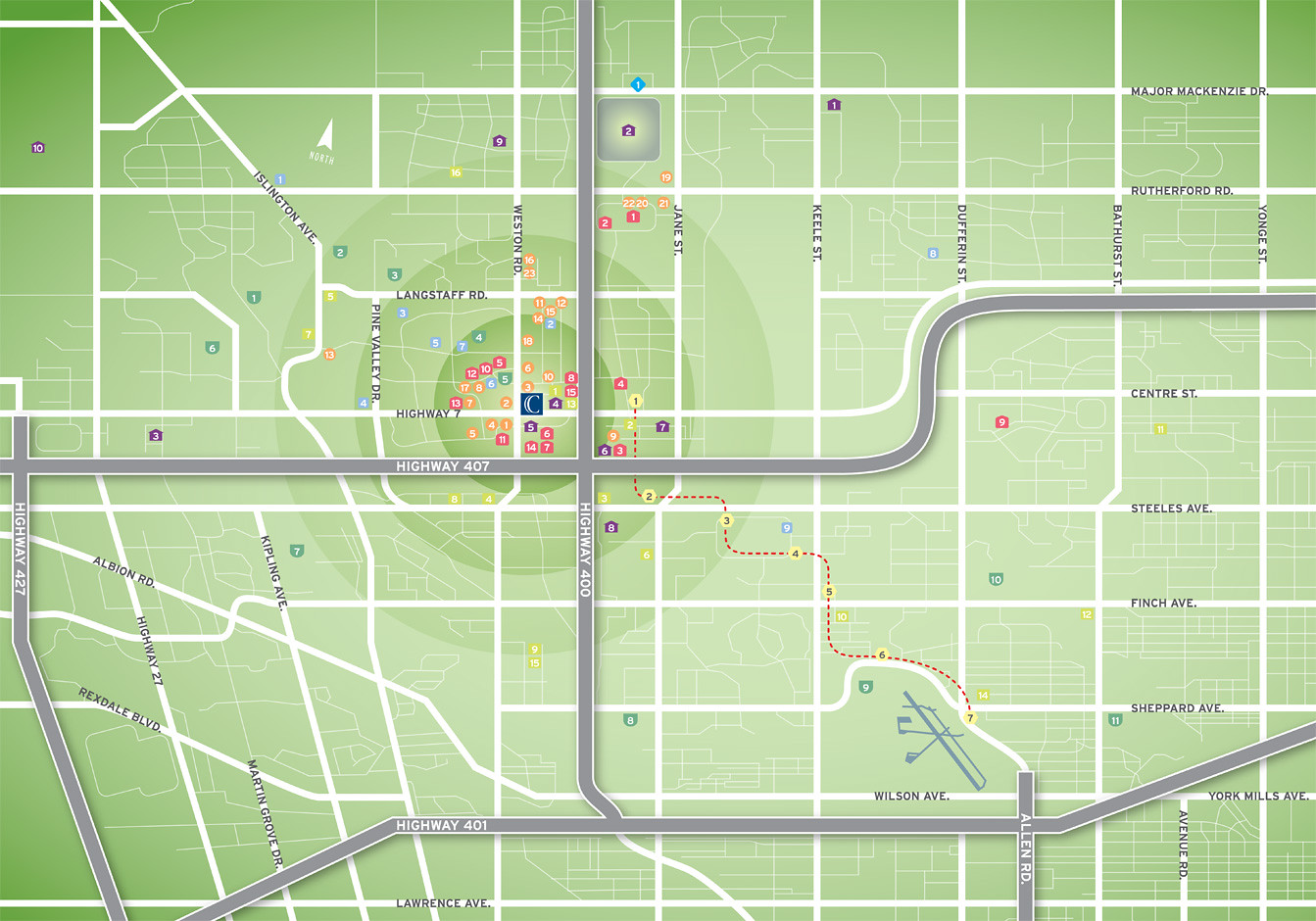The image is a detailed, computerized drawing of a map with a predominantly green background. The map features darker green shading in the top-left, bottom-left, and top-right corners, adding depth to the landscape.

Prominent white lines crisscross the map, representing streets, with thinner white lines indicating smaller roads. Thick gray lines with a white outline highlight major highways, including Highway 407 and Highway 401 running horizontally across the image, and Highway 400 and Allen Road running vertically.

Key streets are labeled, such as Major Mackenzie Drive, Rutherford Road, Centre Street, Steeles Avenue, Finch Avenue, Sheppard Avenue, and Lawrence Avenue, which all run horizontally. Vertically, the map features Weston Road, Jane Street, Keele Street, Dufferin Street, Bathurst Street, and Yonge Street.

At the center-left of the map, three concentric green circles capture attention, populated with numerous small red and yellow icons. A blue icon marked with a large 'C' sits in the absolute center of these circles. Additionally, a dotted red line weaves its way through this central area, adding another layer of detail.